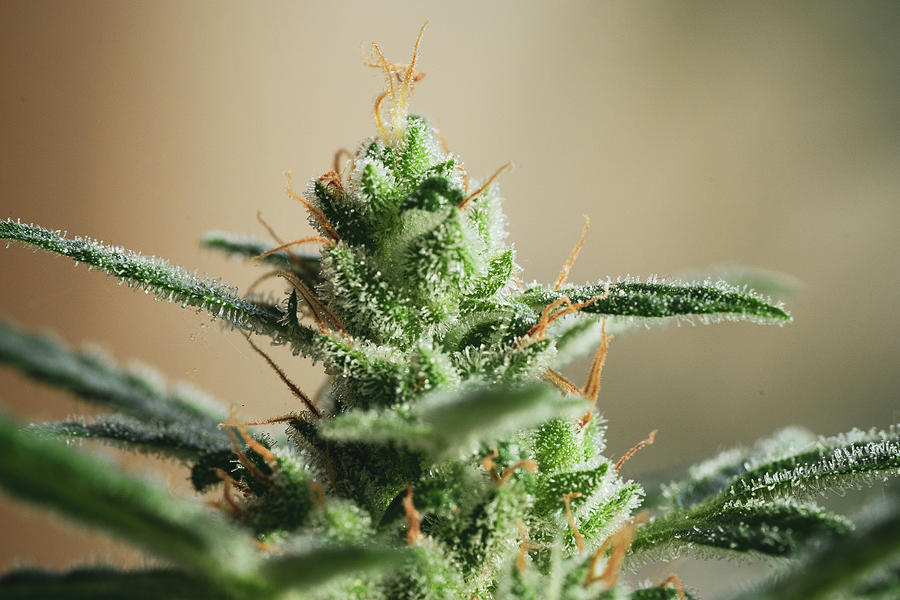This is an extreme close-up color photo of a marijuana bud. The detailed image captures the intricate textures and colors of the plant in striking clarity. The bud itself is predominantly a vivid green, displaying various shades from lighter hues at the top and center to darker tones on the outer leaves. The plant is covered in countless tiny white crystals, suggesting the presence of THC, giving the appearance that it has been dusted with sugar. Interspersed throughout the green and white are numerous tiny, light brown or golden stem-like fibers, known as "hairs," that become darker towards their tips. These fibers appear to emanate from the buds, adding complex texture and color contrast. The background is a highly out-of-focus brown blur, ensuring that all attention is focused on the intricacies of the marijuana bud in the foreground.